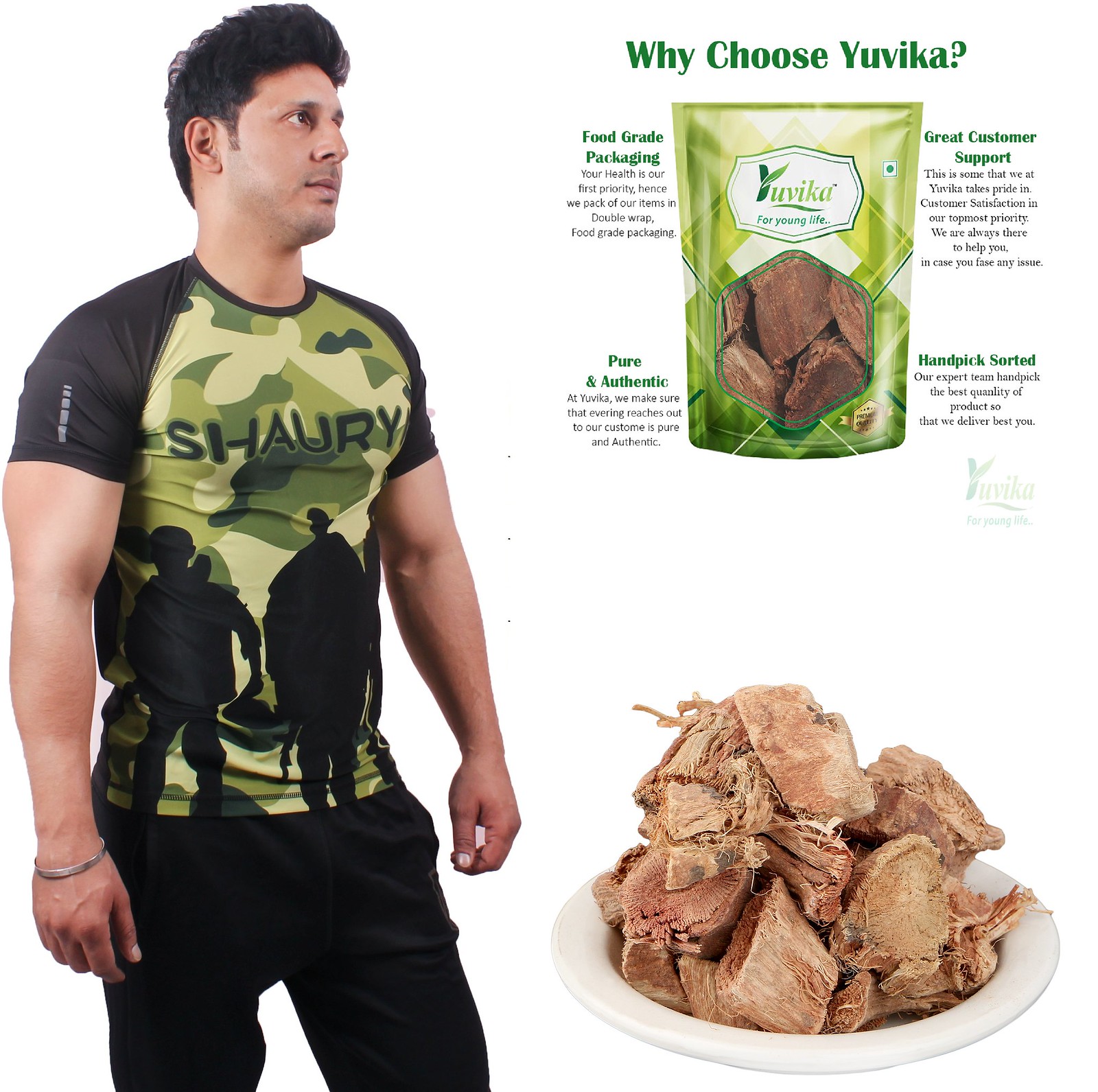The ad features a young man with light brown skin and short, fluffy black hair, standing against a white background. He is dressed in a short-sleeved green camouflage shirt with black sleeves and the word "Shaury" (S-H-A-U-R-Y) printed on the front, accompanied by black outlines of soldiers. He is facing and looking towards the right, with black pants and a bracelet visible.

To the top right of the image, there is a green package containing chunks of meat, labeled "Ukiva." Above the package, in green print, the ad poses the question, "Why choose Ukiva?" and lists benefits such as food-grade packaging, pure and authentic quality, great customer support, and hand-picked, sorted products. Beneath the package, there is a white plate with the meat chunks stacked on it, suggesting the product's appearance. This ad emphasizes the quality and authenticity of Ukiva's meat products, with the young man seemingly contemplating the purchase.